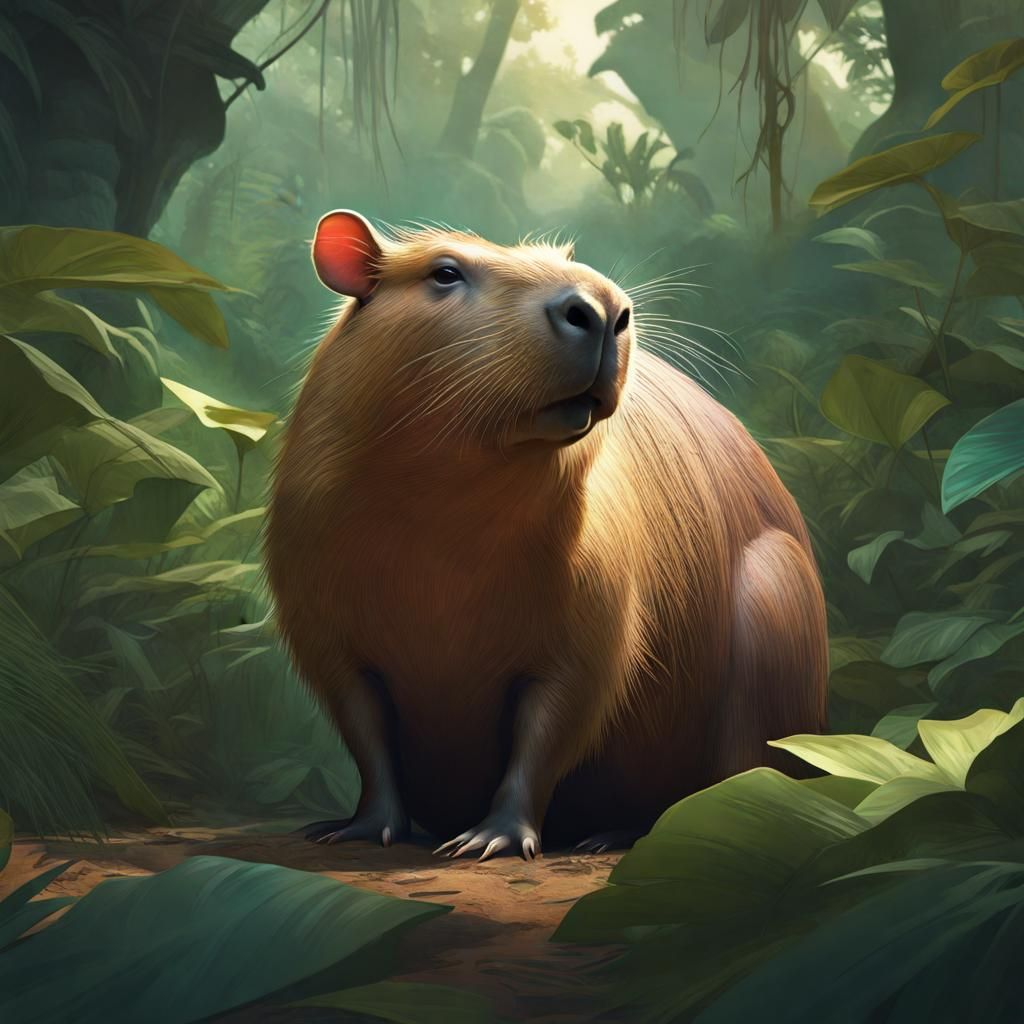This detailed cartoon-like digital image depicts a large capybara prominently positioned in a dense forest setting. The capybara, brown with distinctive whiskers and a notable large nose, stands inquisitively at the forefront. Its fur catches light particularly on the top of the head, right ear, and left shoulder, enhancing its textured appearance. The environment features an array of green leaves, vines hanging from trees, and patches of light filtering through the foliage above. The ground is dirt-colored, marked with footprints likely left by the capybara. The scene, abundant with vines, trees, and various shades of green, provides a tranquil rainforest-like backdrop, suggesting a digitally created or artificially generated illustration.